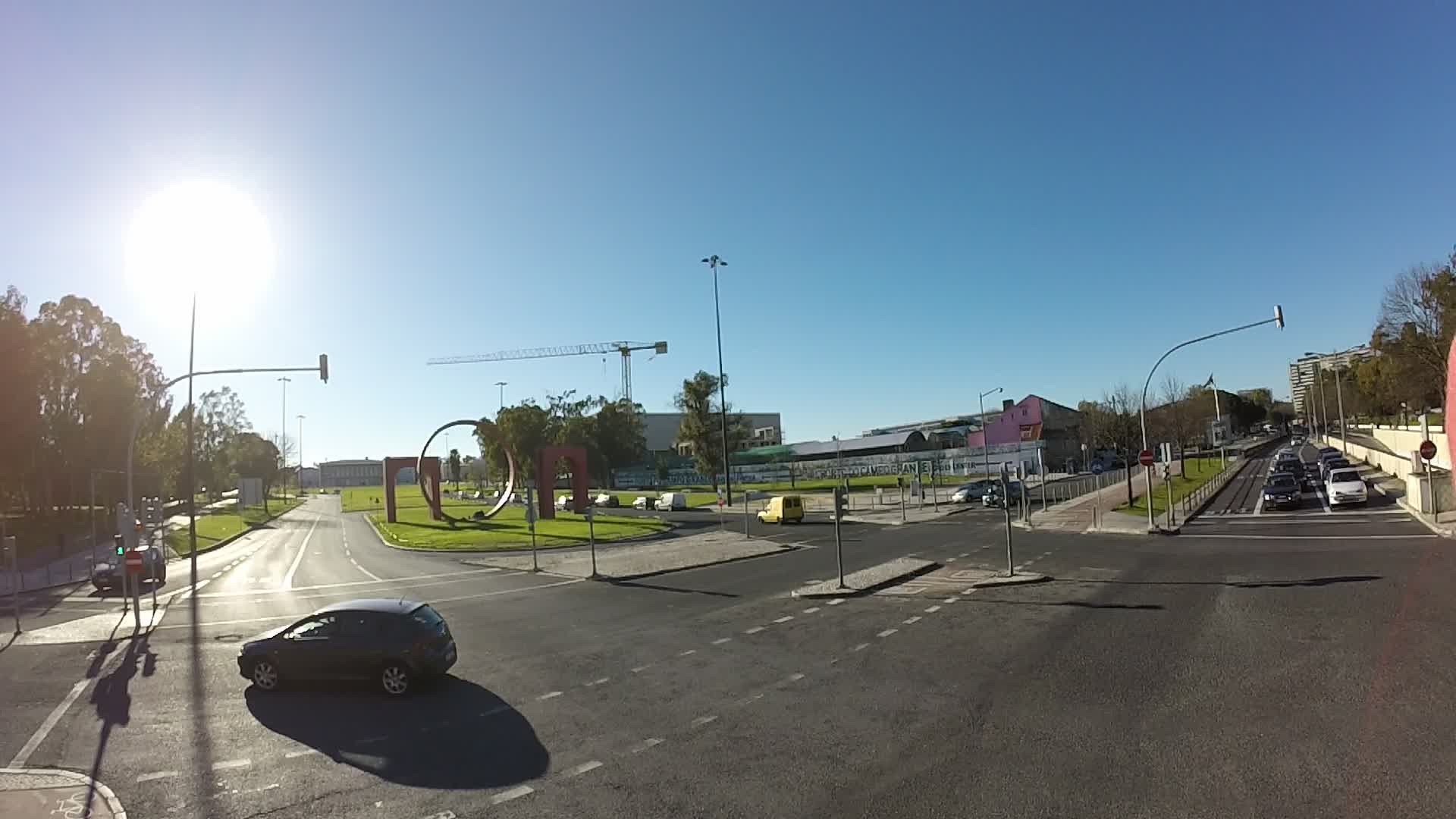This photograph, taken in the afternoon on a bright sunny day with a clear blue sky, captures a dynamic urban scene at an intersection. The sun, a brilliant round orb, dominates the sky, casting sharp shadows and emphasizing the clarity of the day. Straight ahead, cars are halted at a red traffic light, facing a spacious, empty intersection. To the left of the frame, a small compact car is seen maneuvering through a turn into the opposite lane.

Background buildings, suggesting a corporate business district, stand stoically beyond the automobiles, their modern exteriors reflecting a sense of organized urban planning. This district is punctuated with lush greenery and abundant trees, integrating natural elements into the cityscape. Notably, one green space attracts attention with its prominent sculptures: a round circle and two striking red archways, adding an artistic and cultural dimension to the meticulously designed intersection.